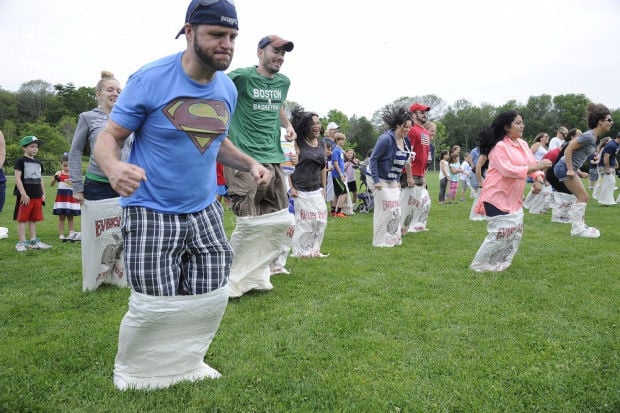This vibrant image captures a lively sack race event in a park, with a group of around 50 to 60 participants hopping energetically on a lush green grassy field. The background reveals a row of green trees and a sky completely covered with gray and white clouds. Everyone involved has their legs snugly tucked into white potato sacks, some of which are adorned with logos.

In the foreground, the focus is on a bearded man wearing a blue Superman T-shirt with the iconic red and yellow emblem, plaid shorts, and a white sack around his legs. He's accessorized with a blue cap sporting sunglasses perched on top, and his facial expression reflects the strain of the race. Just behind him, another tall man smiles broadly, donning a green “Boston” shirt, khaki pants, and a red ball cap. To his right, a tan-skinned woman with long black hair and a peachy pink shirt can be seen energetically participating in the race.

Scattered throughout the scene are other adults, many of European descent with light peach and olive skin tones, adorned in colorful shirts ranging from blue, green, and gray to red. Notably, a man sporting a red shirt and a matching red hat with an American flag is also visible. Behind participants, several children look on intently, cheering for the adults. The image, taken from an angle that provides a right-shoulder view of the competitors, vividly captures the spirit and fun of this community park event.